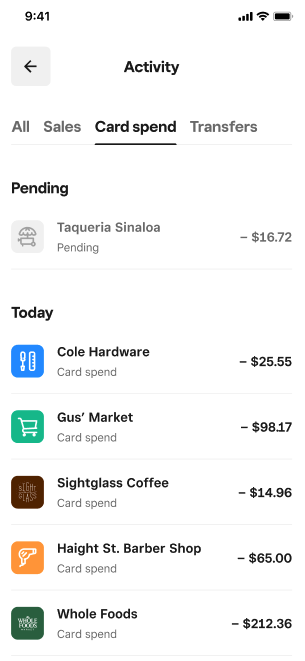This screenshot displays a mobile phone interface at 9:41, showing full service with four bars, Wi-Fi connectivity, and a fully charged battery. At the top left corner, there's a gray box with a black arrow pointing left, labeled "Activities." Below this, there are several menu options including "All," "Sales," and the currently active "Card Spends," indicated by black text while the others are in gray.

Under the "Card Spends" menu, the screen begins with one pending transaction. The section marked "Pending" lists a transaction at Taqueria Sinaloa for $16.72. Following this, a light gray divider separates the "Pending" section from "Today's Transactions."

The "Today's Transactions" section starts with:

1. **Coal Hardware:** $25.55 spent, blue icon.
2. **Gus's Market:** $98.17 spent, green icon.
3. **Site Class Coffee:** $14.96 spent, brown icon.
4. **Haight Street Barbershop:** Spelled "H-A-I-G-H-T," $65 spent, orange icon.
5. **Whole Foods:** $212.36 spent, green icon.

Each transaction is separated by light gray dividers.